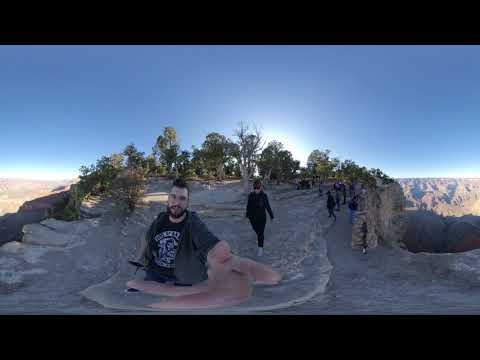In this distorted fisheye lens photo, a young man and a woman are walking on a solid rock walkway atop a mountain, resembling the Grand Canyon's iconic scenery. The man, positioned centrally, has dark hair, a well-kept black beard and mustache, and light-colored skin. He is dressed in a black shirt with some white writing, possibly layered with a dark gray jacket. One of his hands extends towards the camera, its proximity creating a distorted, oversized appearance, with fingers curving backwards. Just behind him to the right, the woman walks forward, clad in a black suit covering her arms and legs, with dark brown hair that falls as she looks downward. Further behind them, the canyon's edges are teeming with people peering over, and lush green trees mark the landscape. The canyon walls exhibit a blend of red and green hues. The expansive sky above is a deep blue without a trace of clouds, and a brilliant white light, likely the sun, illuminates the horizon with a hazy glow. The scene captures a striking high-altitude view down into the vast, shadowed canyon below.